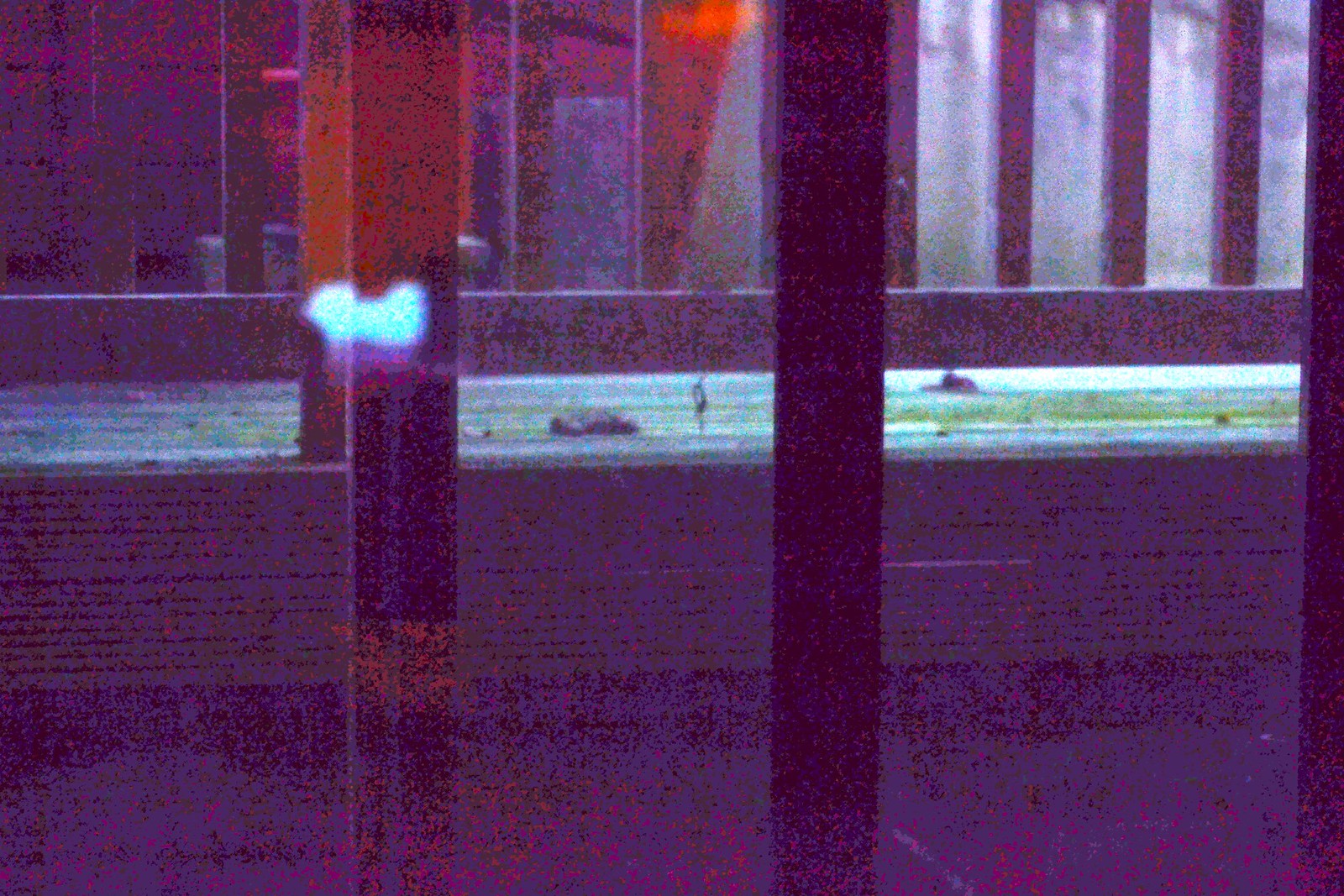This image is a grainy, color photograph or possibly a computer-generated graphic with very low image quality, giving it a blurry and indistinct appearance. The scene is dimly lit, which further complicates the identification of its contents. Vertical, square-shaped black bars span from the bottom to the top of the frame, possibly resembling a railing, sitting on what could be a wooden floor. There's a prominent long, horizontal strip of green in the middle of the image, suggesting a long piece of grass or a running track.

Amidst the dark and grainy setting, there are red patches that look as if they have been screen printed or applied with a paint roller, adding to the chaotic nature of the photograph. In the distance, through a narrow gap between the vertical bars, appears to be a small, white-lit area and possibly a person standing upright on the green strip. Despite the conjectures, the overall scene remains difficult to discern due to its poor clarity and the presence of an ambiguous filter over the image. There are no clear indications of buildings, animals, or vehicles, making the photograph enigmatic and abstract.